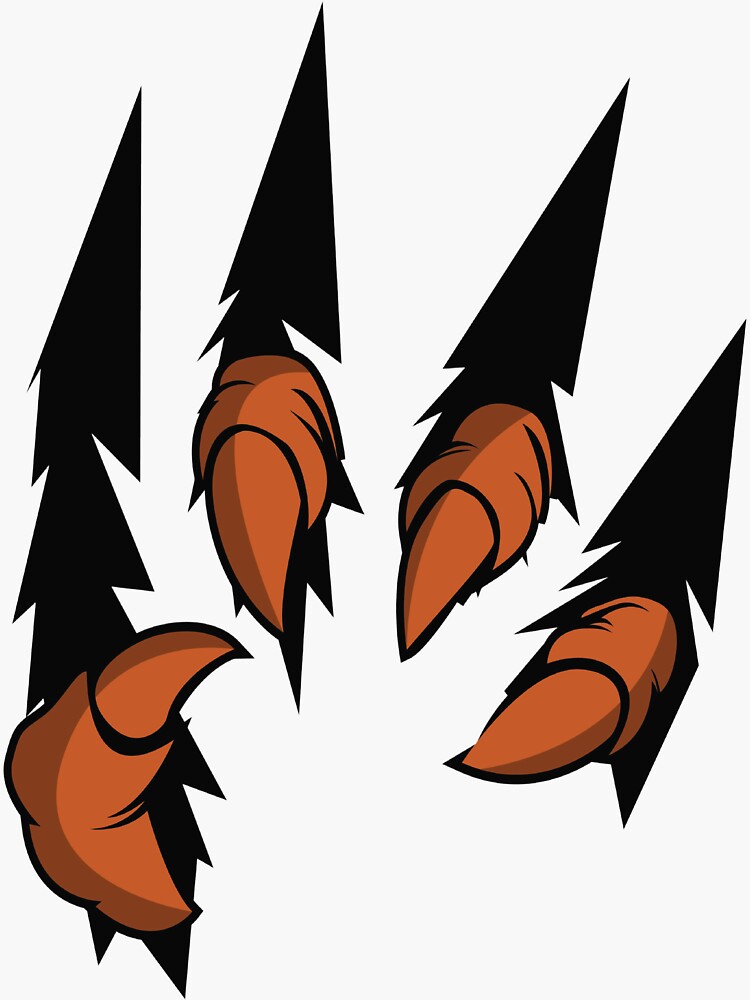The image is a vertical illustration set against a light gray background. It features four jagged, reddish-brown talons or claws, which are intricately detailed with sharp, pointed nails that resemble those of an animal. Each talon appears chunky in shape and the tips are vividly emphasized in orange. Behind each talon are black, arrow-like shapes that point upwards, giving a dynamic, almost lightning bolt effect. The talons are arranged in a semi-circle, and there is no indication of the animal to which these talons belong.